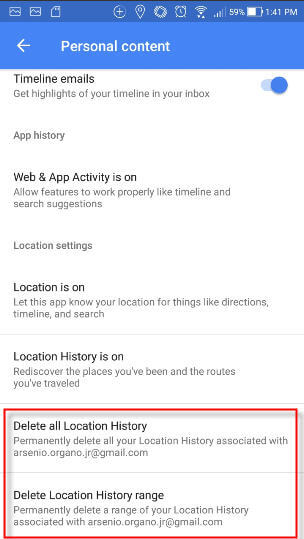The image displays a smartphone screen with a dark blue bar across the top, featuring the usual white icons for Wi-Fi signal, ringer, cellular signal bar, the current time (approximately 1:41 PM), and battery charge at 51%. Just below this bar, there is a blue card with white text, containing some content and an arrow icon pointing to the left and right side of the screen.

The main view of the screen has a white background with black text, detailing several settings options:

1. **Timeline Emails**: "Get highlights of your timeline in your inbox," with a toggle switch that can be slid to the left to turn off or to the right to turn on.

2. **App History**: Listed below is the option for Web and App Activity, currently marked as "On." This setting allows features like Timeline and Search Suggestion to work properly.

3. **Location Settings**:
   - "Location is On," enabling the app to use your location for features like Directions, Timeline, and Search.
   - A separating line followed by "Location History is On," which helps to rediscover places you've been and routes you've traveled.

At the bottom, within a red-outlined rectangle, there are options for:
- "Delete all location history": Permanently delete all location history associated with the email Arsenio.Morgano.Jr@gmail.com.
- "Delete location history range": Permanently delete a specified range of your location history associated with the email Arsenio.Morgano.Jr@gmail.com.

This detailed caption effectively describes the smartphone screen's layout and each element's functionality, giving a comprehensive view of the display and settings.